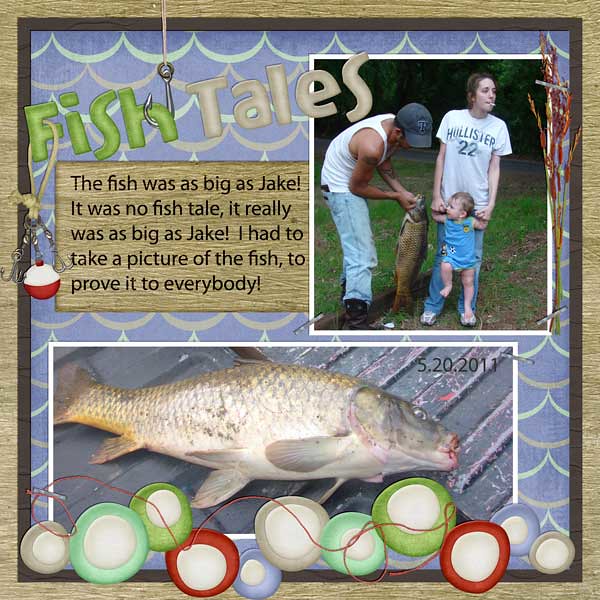The image depicts a card with a wooden, brownish border. Dominating the scene is the playful title "Fishtails," emphasizing the word "fish" in green and "tails" in light gray. The word "fish" is intertwined with a fishing hook that extends from the top left, curling beneath the H. A red and white bobber dangles from the uppercase F, reaching down to the middle left of the card. Adjacent to the bobber, a rectangular panel with a wooden background contains five lines of black print.

To the right of this panel, a photograph captures a family moment: a man holding a large fish, a woman in a white t-shirt holding a child clothed in a blue onesie. The child is captivated by the fish. The lower portion of the card features another fish image stretched diagonally, accompanied by the date "5-20-11-2011." Below this image, an array of colorful circular designs, resembling bobbers, runs along the card's base. This lively and detailed composition celebrates the family's fishing adventure, humorously asserting, "The fish was as big as Jake. It was no fishtail. It really was as big as Jake," ensuring proof of their impressive catch.